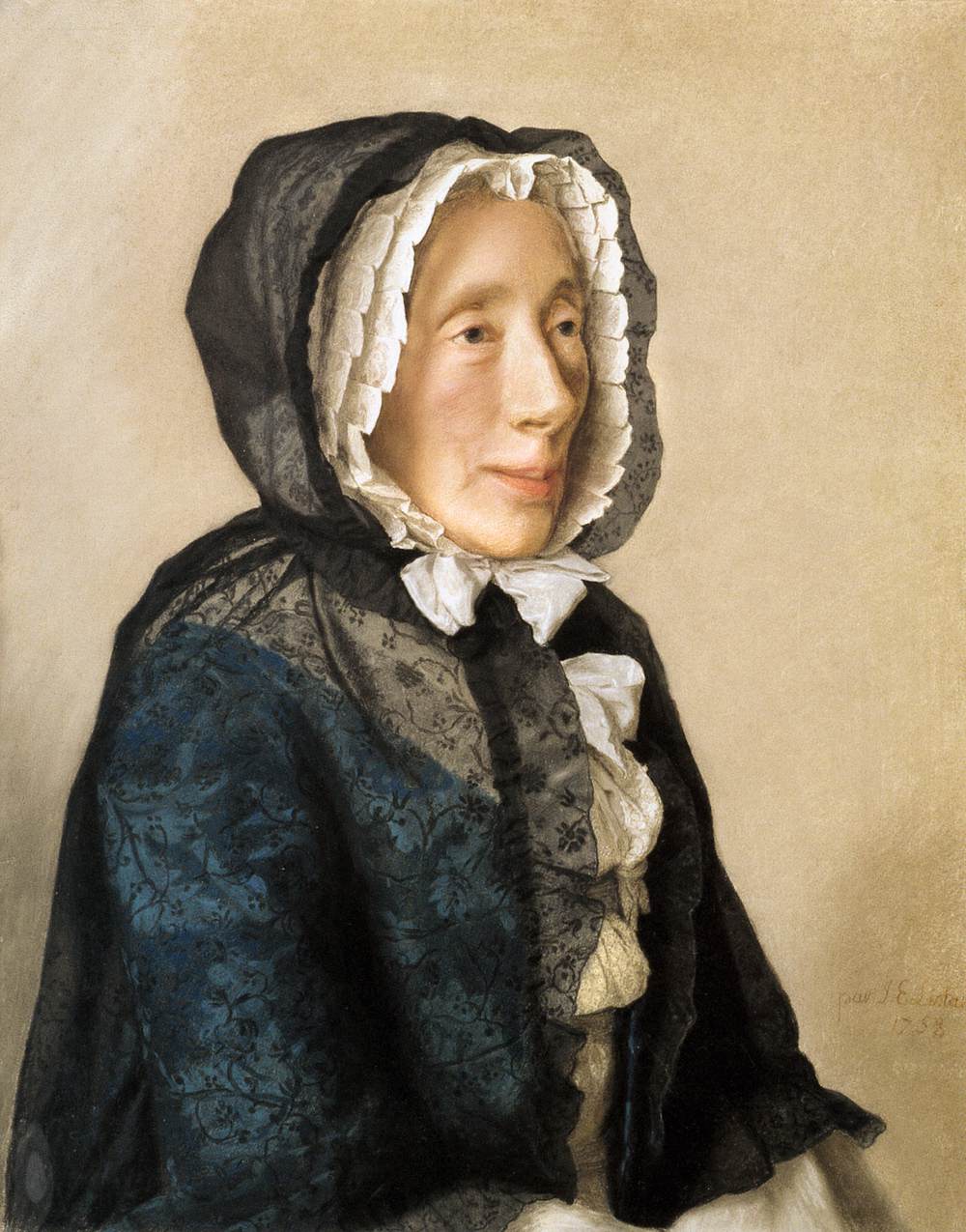This is a detailed oil painting from 1758 by Jean-Étienne Léotard, titled "Madame Jean Trochin." The portrait features an older woman seated and depicted from the waist up, positioned towards the left side of the image with her gaze directed slightly upward to the right, presenting a pleasant half-smile. She is dressed in a distinctive black lace jacket that is semi-transparent, adorned with intricate patterns, and includes a hood that drapes over her head. Beneath this, she wears a ruffled white bonnet, tied in a bow at her neck, with visible ruffles cascading down her chest. Her attire also includes a blue dress underneath the jacket. The background is a plain beige, enhancing the focus on the subject. The artist's signature and the creation year, 1758, are subtly noted in the bottom right corner of the painting.